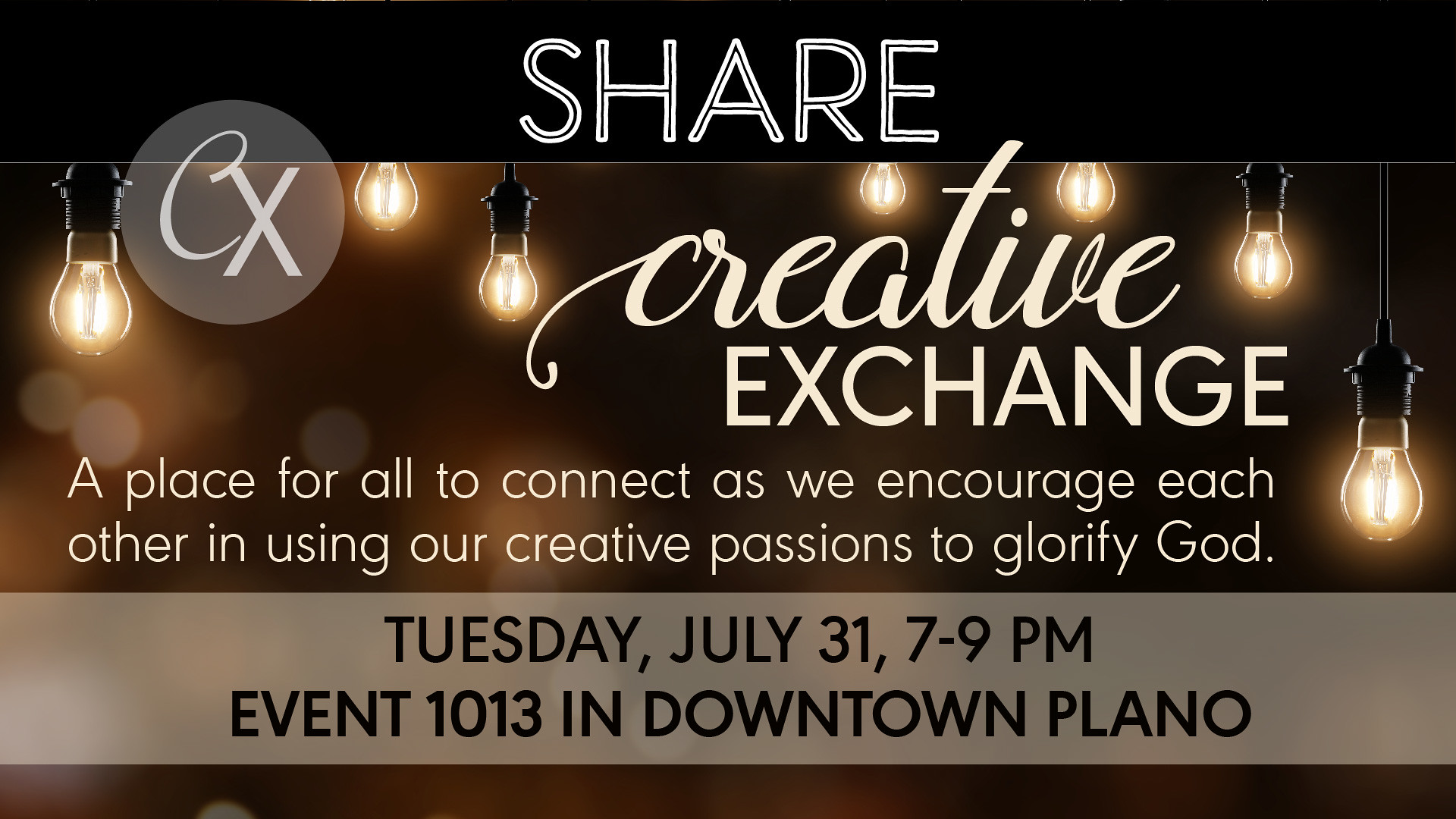The image is an advertisement for an event featuring a vertically oriented flyer with a distinct black header at the top. The text on the header reads "Share." Below this, the background transitions to a brown hue adorned with soft-focus circles of amber light, enhancing the warm and inviting atmosphere. Hanging from the top are glowing light bulbs on black cords, adding to the decorative element. Dominating the center is the text "Creative Exchange," followed by the tagline "a place for all to connect as we encourage each other and use our creative passions to glorify God." Toward the bottom, against a gray background, essential details about the event are clearly presented: "Tuesday, July 31st, 7-9 p.m., Event 1013, in downtown Plano." Additionally, on the far left side of the flyer, there's a semi-transparent circle with the initials "CX," further branding the event.